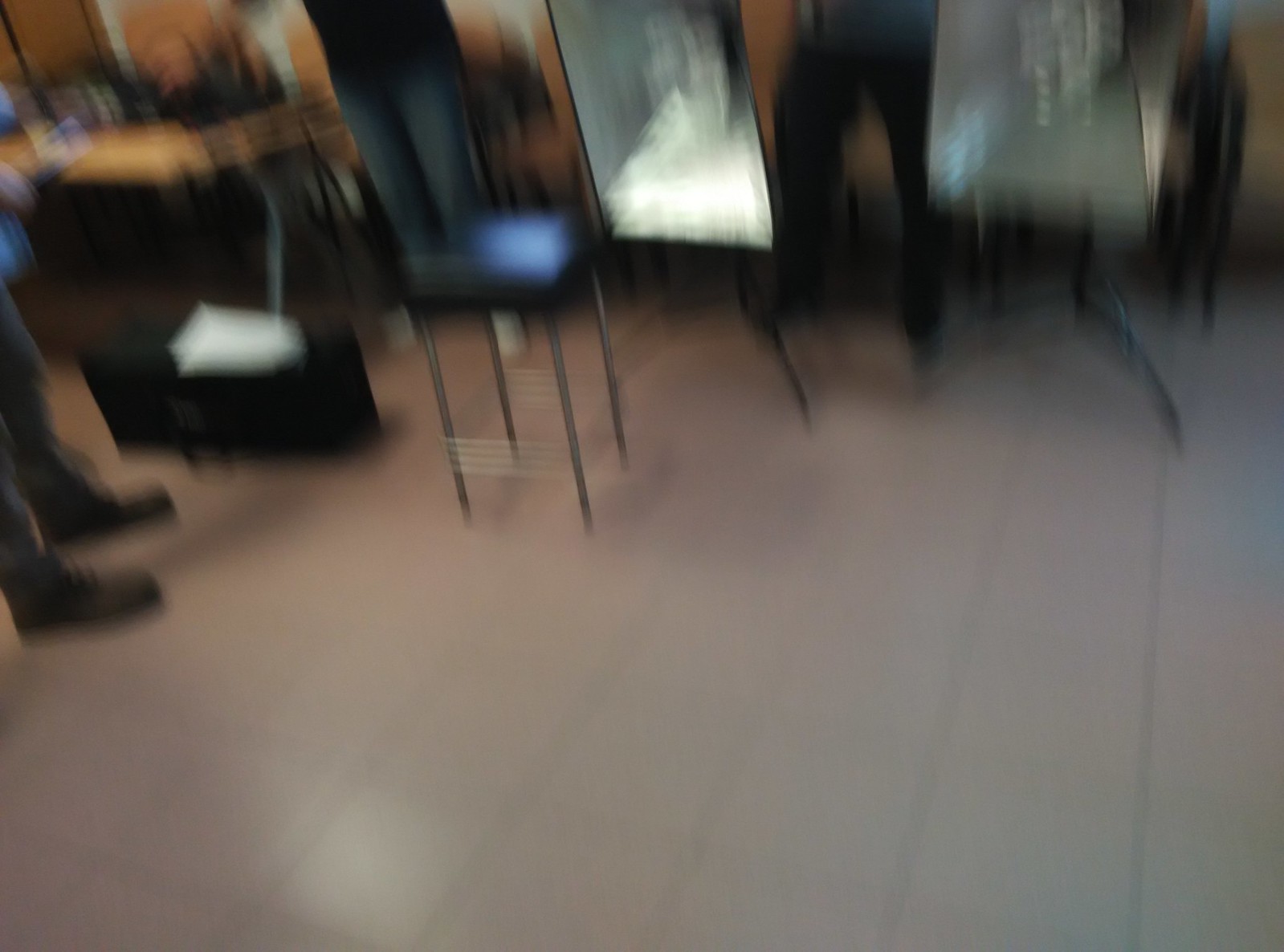The image depicts the interior of a room with a white tile floor. The photograph is extremely blurry, making specific details challenging to discern. Central near the front, there is a chair with long silver legs and a black cushion. To the left of the chair, there are two free-standing mirrors, one directly to the left and another to the right, both with black outlines. Behind the mirrors, a wooden wall is visible. A table with multiple bottles is positioned to the far left. Additionally, two pairs of legs with brown shoes and dark pants, possibly blue jeans, are partially visible in the lower left corner of the image. The overall scene appears to be an indoor setting, potentially an office, a shopping area, or a coffee shop.